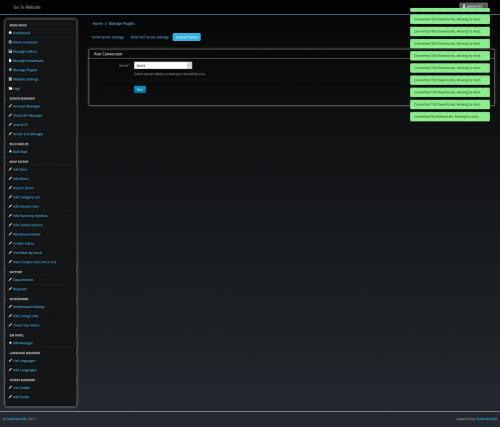The image features a black square with an abundance of minuscule text, making it challenging to discern the website's nature. In the top left corner, there's some text, but its diminutive size renders it unreadable. Running vertically along the left side of the image are several clickable options, identifiable by their blue text and accompanying icons; however, the text is too small to be legible. At the top center of the image, there are additional selectable options, equally difficult to read. In the top right corner, there are approximately 9 to 10 light green tabs, each containing text that similarly suffers from being too tiny to decipher.